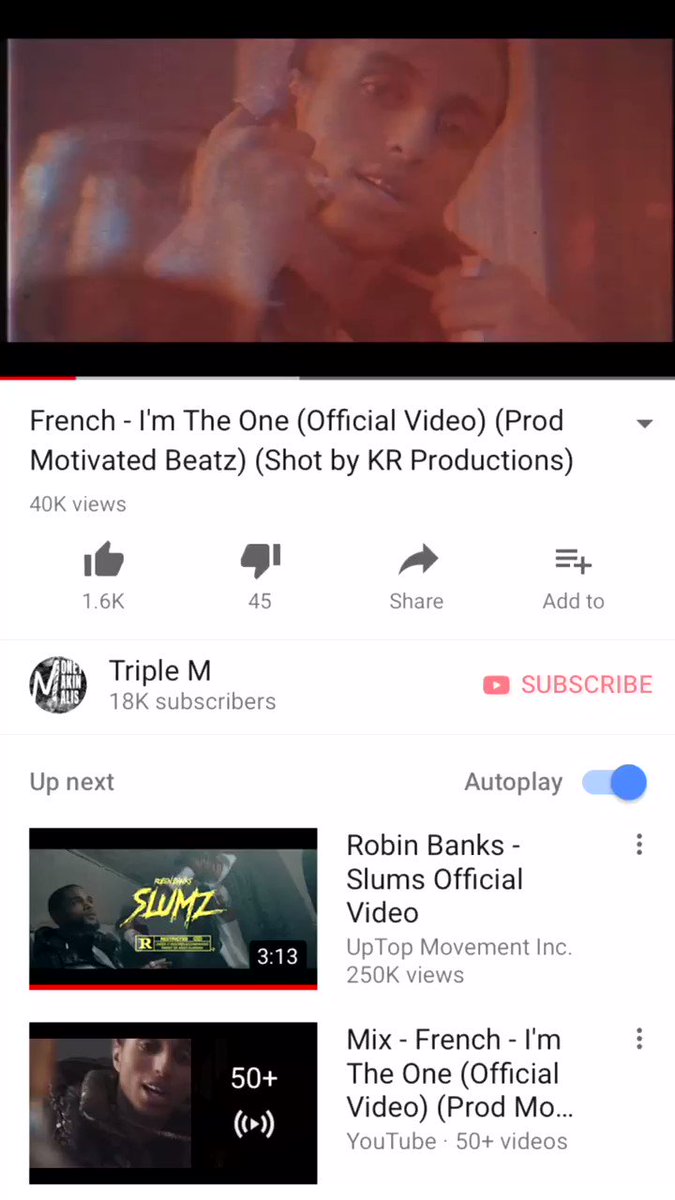Image Description: 

The image displays a smart TV screen showcasing a YouTube video. The current video being played is titled "French, I'm the One, Official Video." The screen features a headshot of a Frenchman, framed within dark, moody colors including reds and browns. The man's face is clearly visible, along with both of his hands.

The footage is bordered by black bars at the top and bottom of the screen. On the bottom bar, text indicates that the video is "Shot by KR Productions" and "Product Motivated BEATZ." The video has garnered 40,000 views.

Below the video, the YouTube interface shows the channel "Triple M," which has 18,000 subscribers. Next to the channel name, a red "Subscribe" button appears. Beside this button, there's a round black and white icon displaying an "M" in the center.

On the right side of the screen, under the "Up next" section, there's another video thumbnail. This thumbnail shares the same rated R branding and previews a runtime of 3 minutes and 13 seconds. The text accompanying the thumbnail mentions "Mix French: I'm the One, Official Video" produced by "MO." This video is also noted to be part of a playlist, indicated by the tag "YouTube 50+," and it features the same image of the man from the currently playing video.